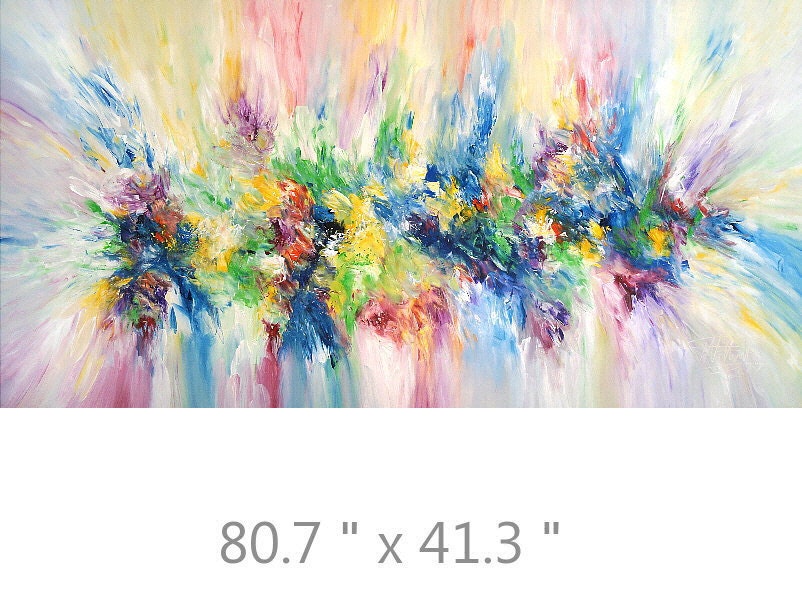This captivating abstract painting, measuring 80.7 inches by 41.3 inches, boasts an intricate and vibrant composition that draws the viewer's eye to its center. At the heart of the artwork, thick splotches of paint in a multitude of colors, including blue, yellow, pink, red, green, dark blue, and dark red, merge together in a blurred, impressionist style, evoking the image of a lively bouquet of flowers. From this colorful epicenter, the hues gradually fan out towards the edges of the canvas, transforming into delicate, feathery brushstrokes with a softer, watercolor-like appearance. The pastel shades and dynamic brushwork create a rhythmic flow across the rectangular canvas, making it a stunning piece that would likely be featured in an art catalog and ideal for wall display.